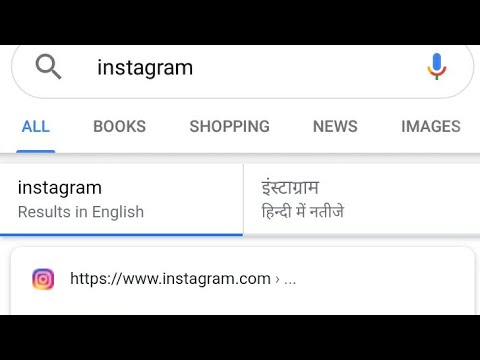This image is a screenshot of Google search results for the term "Instagram." The interface suggests it might be the Google app, as indicated by the prominently visible small microphone icon. The search box at the top contains the recognizable search icon alongside the text "Instagram." The webpage is predominantly white with black font and some blue-highlighted words.

Directly beneath the search box, the "All" tab is highlighted, with adjacent tabs for "Books," "Shopping," "News," and "Images" extending to the right. Following this navigation bar, another horizontal bar displays the text "Instagram results in English," accompanied by what appears to be Mandarin characters and a checkbox indicating the original language of the search results. The primary search result showcases Instagram's logo and presents a clickable link to "www.instagram.com." The screenshot does not extend further down the page, focusing solely on these elements.